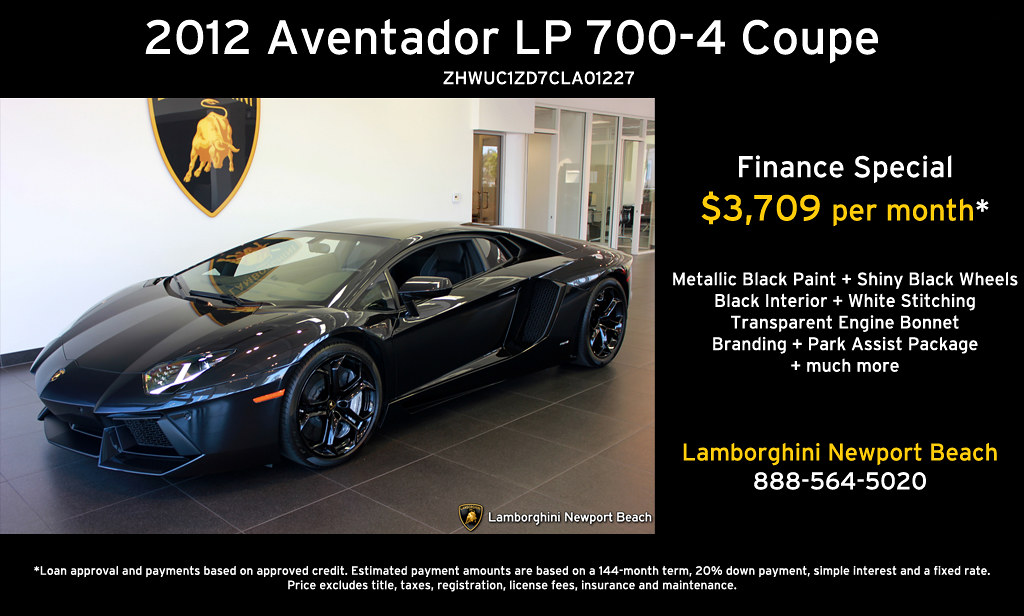This photograph shows a detailed advertisement for a Lamborghini Aventador LP700-4 Coupe on display at the Lamborghini Newport Beach dealership. The central focus of the image is a sleek, dark gray Lamborghini with a transparent engine bonnet and shiny black wheels, positioned horizontally within a showroom setting. The car, featuring black interior with white stitching, is angled to the left, facing the viewer.

The background is a black poster with white and yellow text. At the top in bold white letters, it states "2012 Aventador LP700-4 Coupe," followed by the vehicle's VIN number. On the right side, also in white letters, it highlights a "Finance Special" for $3,709 per month. Below this, the details of the car’s features are listed in smaller white text: metallic black paint, shiny black wheels, black interior, white stitching, transparent engine bonnet, and a branding and park assist package.

In yellow letters, the advertisement prominently mentions "Lamborghini Newport Beach" along with the dealership's phone number. The lower border of the image contains additional fine print detailing loan approval and payment terms: "Payments based on approved credit, estimated payment amounts based on a 144-month term with 20% down, simple interest, and a fixed rate. Price excludes title, taxes, registration, license fees, insurance, and maintenance." The Lamborghini emblem, a bull within a shield of gold, is visible on the white wall behind the car, reinforcing the brand's luxury and status.